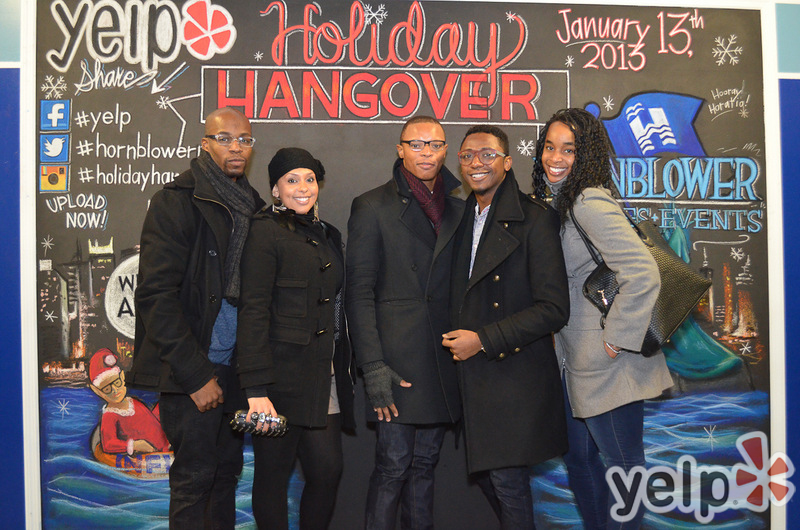The image captures a group of five Black individuals standing together in front of a promotional sign for a Yelp event. Behind them, a black chalkboard prominently displays a chalk-written “Yelp” and several social media indicators, including the Facebook, Twitter, and Instagram logos with hashtags like #Yelp, #Hornblower, and #HolidayHangover. Instructions to “upload now” are also visible. The event is titled "Holiday Hangover," which is dated January 13, 2013. On the chalkboard, near the bottom right corner, a faint Yelp logo can be seen.

Starting from the left, the first person is a Black man dressed in a blue top, black scarf, black coat, and black trousers, wearing black-framed glasses. Next to him is a Black woman in a black coat, black tights, and a black hat, holding a purse and adorned with large rings on her fingers. The middle individual is a Black man wearing a red scarf, black coat, black fingerless gloves, black jeans, and black-framed glasses. To his right is another Black man with shaved hair, red-framed glasses, a white shirt, and a black coat. The last person is a Black woman with long curly hair, wearing a grey jacket, blue jeans, and carrying a large black bag over her shoulder.

All five are looking directly at the camera; some are smiling while others are not. The scene appears to be from a colder day or evening, as they are all dressed in jackets.